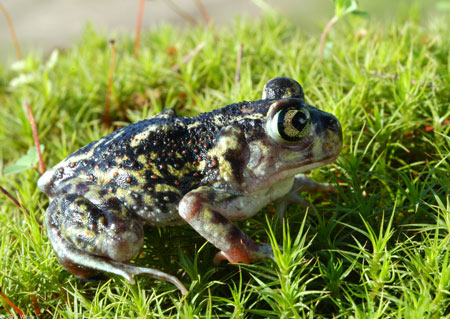The image captures a close-up of a frog, centrally positioned with its head slightly to the right. The frog's body displays a rough texture with a mix of slimy, yellowish-green coloration and prominent black markings along its back. Interspersed within these black portions are small spikes or bumps on its skin. The frog’s large, yellow eyes with dark, rounded centers protrude noticeably from its head. Its underbelly, which peeks out slightly, is of a lighter, tan hue. The frog rests on short grass that gently slopes, with the right side appearing marginally taller than the left. Brownish twigs poke out from the grassy patch, and dark soil is visible beneath the vegetation.